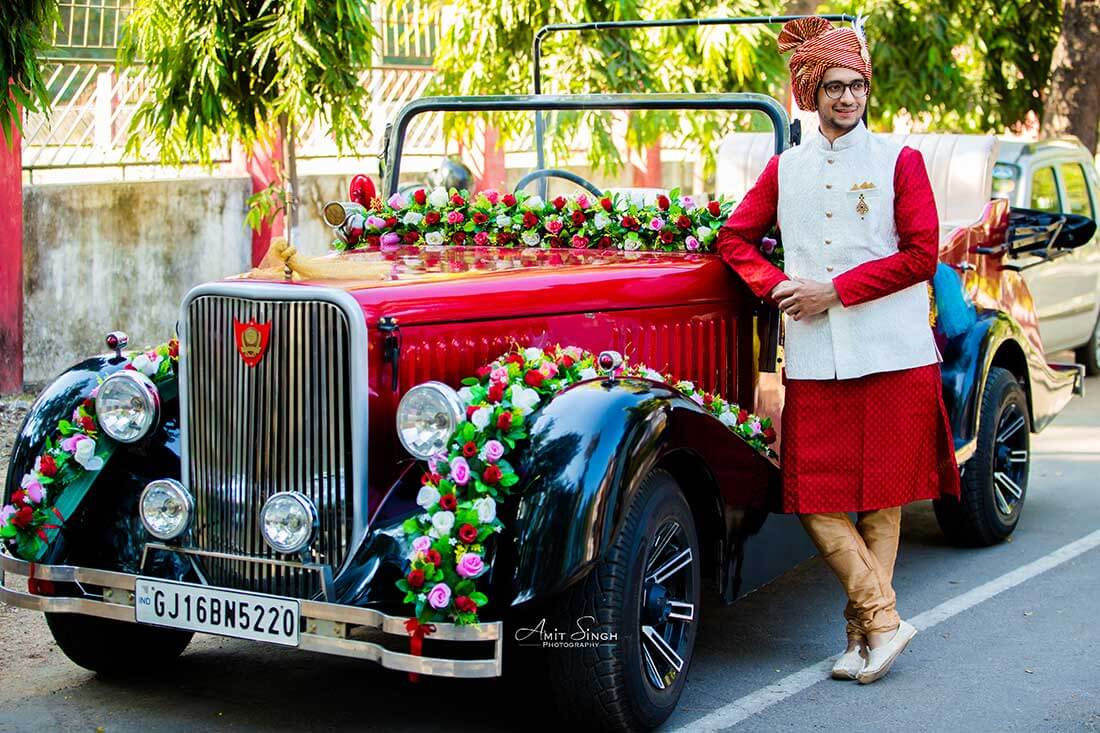A color photograph depicts a man posing with a parked, antique-style convertible car, reminiscent of the 1940s, featuring a shiny red body and black trim. The car is adorned with red, pink, and white flowers, with green leaves hanging around the top. It also has a silver radiator with a red badge and large black rims over the front tires. A white license plate reading "GJ16BN5220" is prominently displayed in the front. The man, leaning against the vehicle with his right elbow on the hood, is dressed in a culturally inspired outfit that includes a long-sleeved red shirt extending to his knees, brown leggings, white shoes, and a white, sleeveless button-up vest. He also wears a red and white turban-like headdress. In the background, there's a dirty cement wall, a parked white car, and trees lining the street.